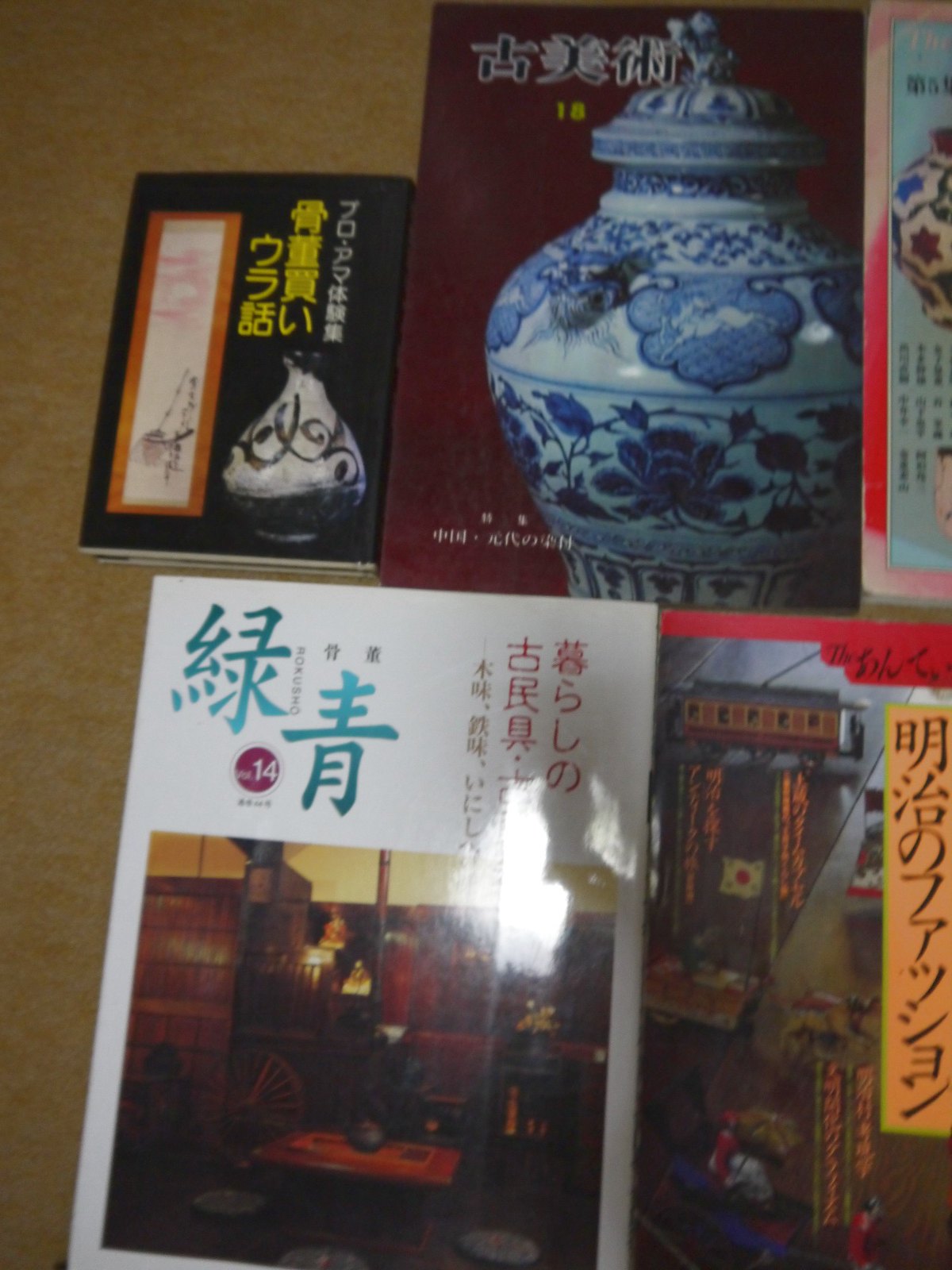This image captures an assortment of five Japanese books laid out meticulously on a flat, orangish-brown surface, viewed from above. The books' titles are vertically aligned and presented in various colored kanji, contributing to a visually striking arrangement against the background. The top left book features a black cover adorned with a black-and-white photograph of a vase, suggesting a focus on pottery. Adjacent to it, another book showcases a large blue-and-white ginger jar, accentuating its detailed ceramic design. To the right, a sliver of the third book hints at another pottery form. Below these, the bottom row includes a book with a glaring light reflection on its cover, obscuring the details but revealing some color photography. In the bottom right corner, the final book, which also stands vertically, is partially obscured but hints at traditional architectural imagery or street scenes. The creamy yellow wall in the background highlights the books and vase, adding a warm ambiance to the captured still life.